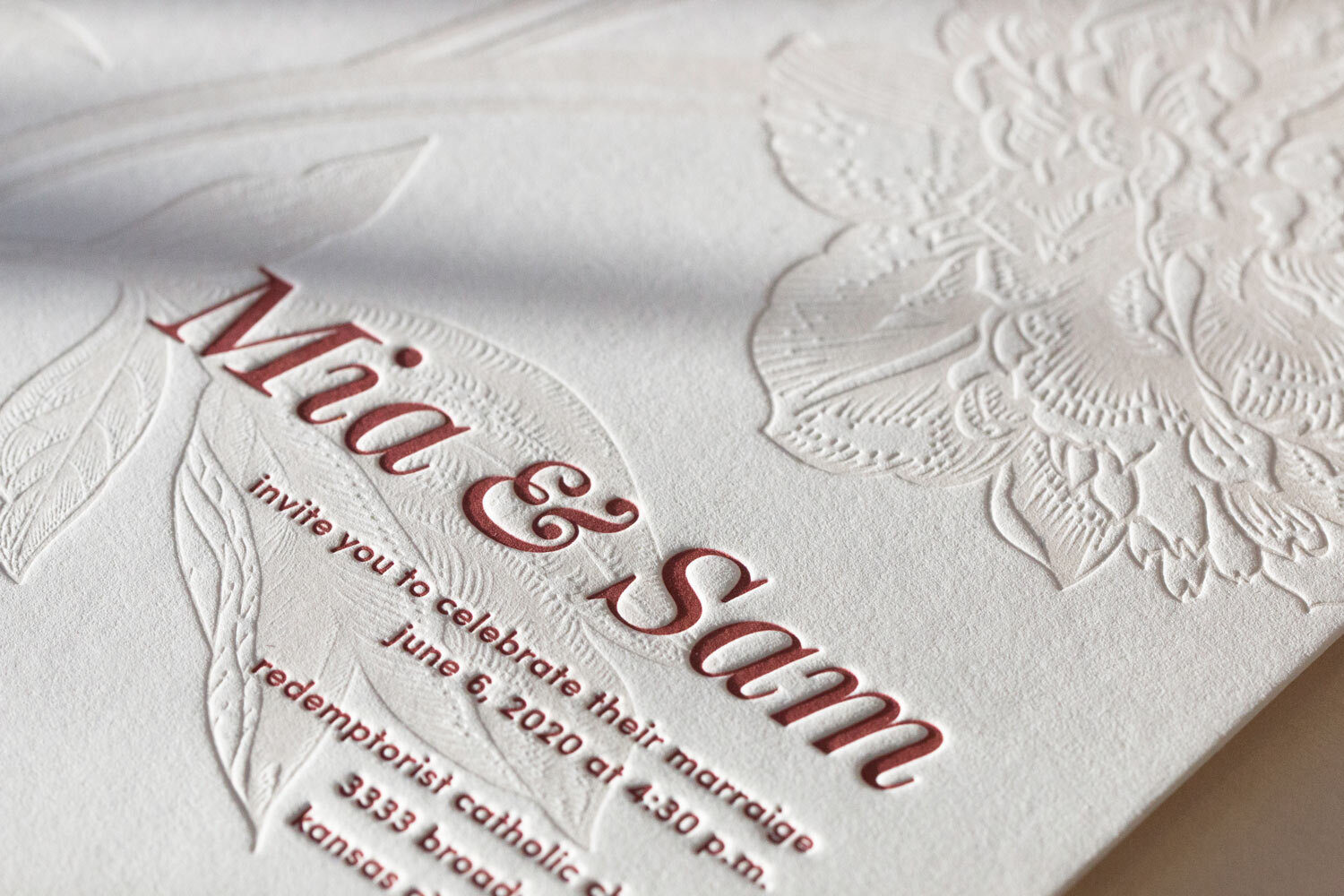This detailed photograph showcases a wedding invitation card prominently featuring red Arial font on a thick white background. The card invites guests to celebrate the marriage of Mia and Sam on June 6, 2020, at 4:30 PM. The text below specifies "Redemptorist Catholic," indicating the ceremony's location, though the full address is partially obscured, revealing only "3333" and "Kansas." 

The card is presented diagonally, with its top angled toward the top right of the image. The design is beautifully adorned with embossed floral motifs, including pleated roses and what appear to be daffodils, with intricate petals slightly out of focus, lending a delicate, lacy aesthetic. The main focus is on the celebratory text "Mia and Sam" and their wedding details, highlighted against the elegant textured backdrop.